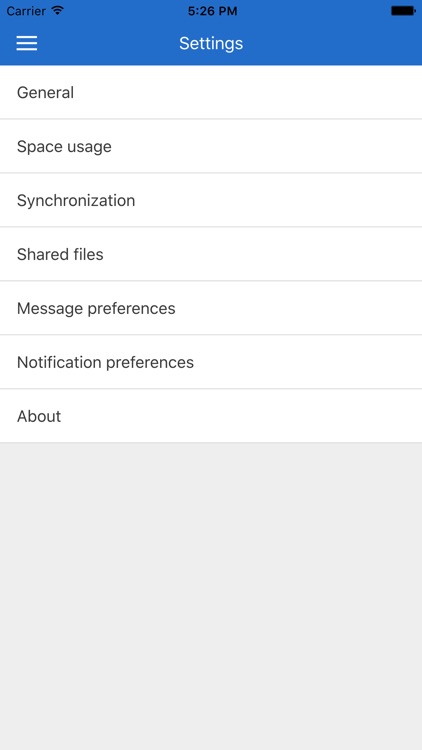The image is a screen capture from a mobile device, showcasing the device's "Settings" menu. At the top of the screen, a blue bar spans horizontally, and within it, the following details are visible: on the upper left, the word "carrier" is written in black text; in the center, the current time "5:26 p.m." is also displayed in black; and on the upper right, a battery icon indicates the device's battery status. Directly below the blue bar and centered on the screen, the word "Settings" is prominently displayed in white text.

The main content of the screen features a list of setting options arrayed vertically on the left side, each setting presented in its own row with a gray horizontal line separating them. The settings, listed from top to bottom, include:

1. **General**
2. **Space Usage**
3. **Synchronization**
4. **Shared Files**
5. **Message Preferences**
6. **Notification Preferences**
7. **About**

Following the "About" option, there is a blank gray rectangular area devoid of any text or icons, completing the visual structure of the device's settings menu.